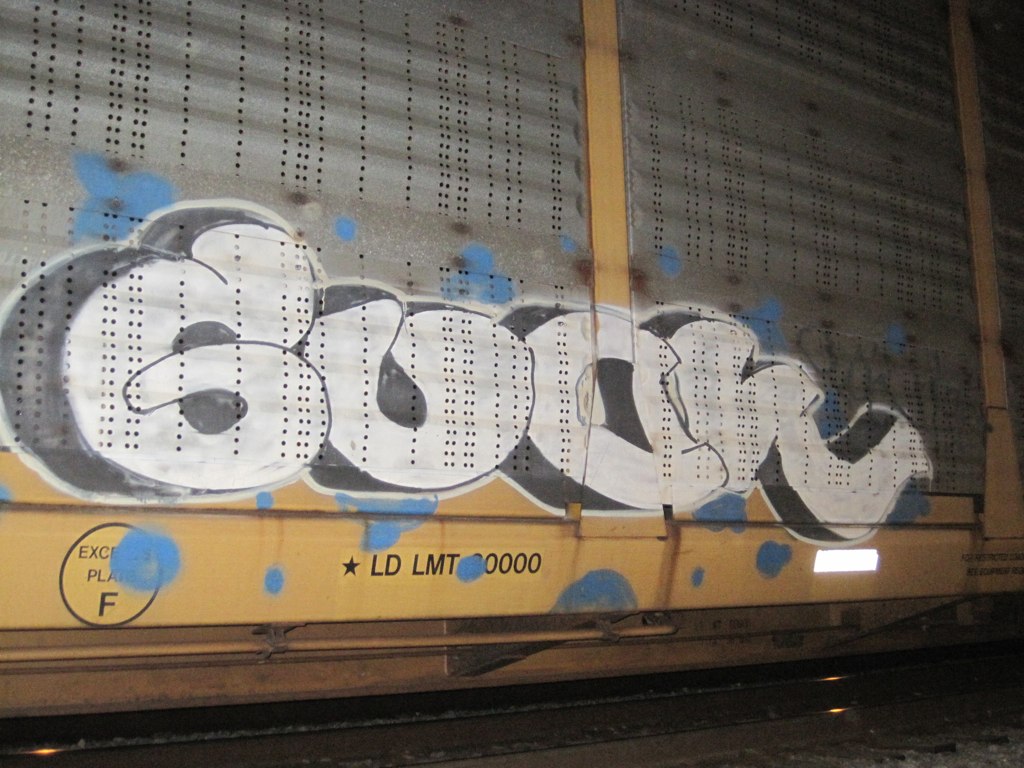The image features a detailed side view of a gray cargo train, constructed from steel plates that are punctuated by rows of small holes. These holes suggest that the train might be used for transporting livestock, perhaps horses. The train features a mix of colors, notably gray with some yellow steel plates visible as well. At the bottom of the train, there is a reflector. Scrawled across the train's side is prominent white graffiti with black shadows accented by sporadic blue splotches. Text on the train includes "LDLMT" followed by four zeros (0000), and there is a circular marking with a black letter "F" on it. The combined elements of color, text, and graffiti create a visually complex and textured image.